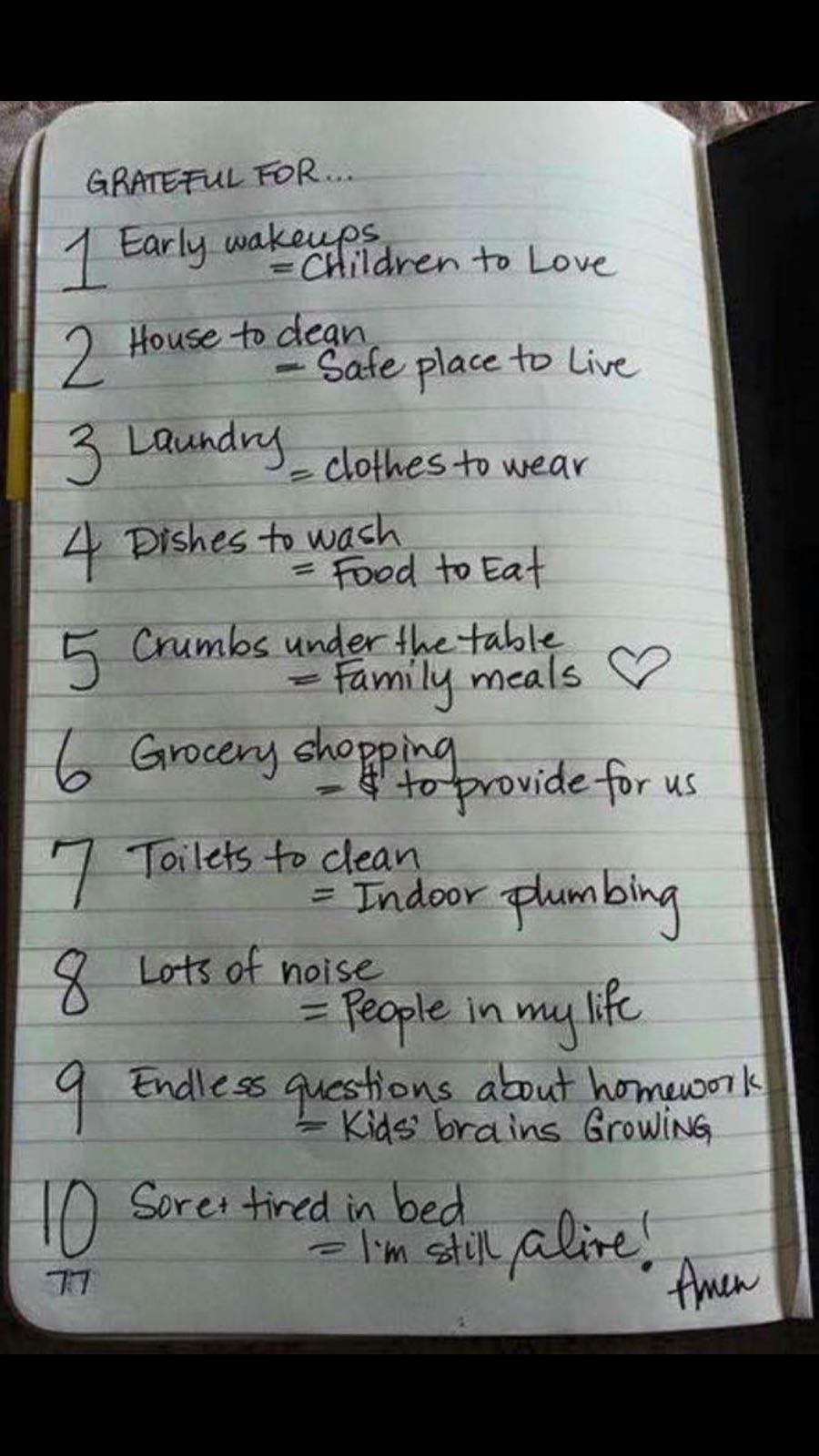In this color photograph, taken in portrait orientation, we see a single central object—a notepad occupying nearly the entire image with black borders at the top and bottom. The background is dark, setting a focused indoor atmosphere. The white pages of the open notepad feature horizontal ruled lines and are written on in black ink. At the top of the page, it reads "Grateful For..." followed by a list numbered one through ten, with each entry spaced across two lines. The handwritten gratitude list begins with "Early Wake-Ups = Children to Love" and continues with items like "House to Clean = Safe Place to Live," "Laundry = Clothes to Wear," and "Dishes to Wash = Food to Eat." Mid-list, a hand-drawn heart emphasizes "Crumbs Under the Table = Family Meals." Further down, practical gratitudes such as "Grocery Shopping = Dollars to Provide for Us" and "Toilets to Clean = Indoor Plumbing" are noted. The list concludes with "Lots of Noise = People in My Life," "Endless Questions about Homework = Kids' Brains Growing," and "Sore and Tired in Bed = I'm Still Alive." Under the final entry, the number "77" and the word "Amen" appear in the lower right-hand corner, suggesting a reflective and personal touch to the gratitude journal entry. The notepad's central, prominent positioning and the detailed realism of the photograph effectively convey a meaningful message of appreciation for everyday tasks and moments.